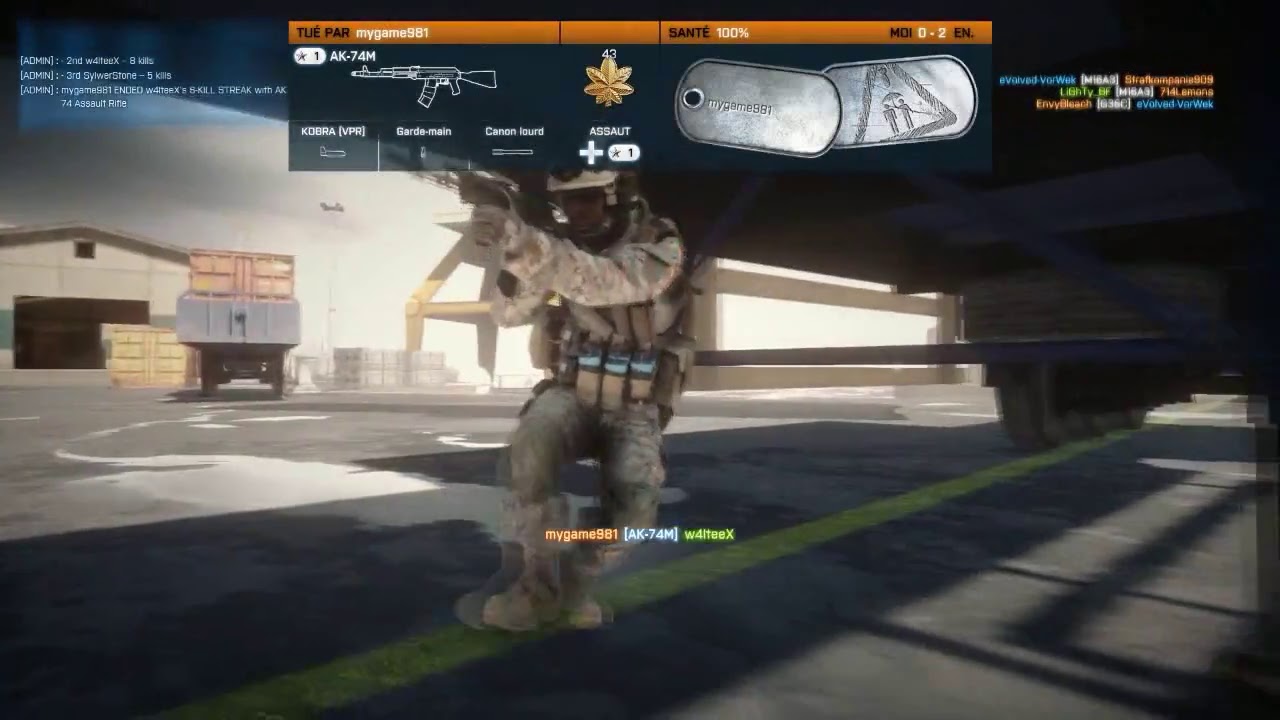This detailed screenshot from a computer war game captures a dynamic military scene on a base. Dominating the center of the image is a soldier clad in brown and white camouflage, emerging from a vehicle and stepping onto a paved road marked with a yellow line. The soldier, positioned directly in the middle, is pointing forward with an AK-74M rifle; his gun and tactical gear prominently displayed, including various pouches around his waist. He wears a white helmet and appears to be fully equipped for combat.

The setting, an outdoor military zone, is bathed in daylight. To the left, there is an open warehouse with additional shipping containers scattered around, and a truck with a loaded shipping container parked in front of it. The background features a hangar and other military vehicles, with an aircraft seen flying in the sky. 

Additional details include an orange banner at the top displaying names and statistics like "2PAR," "my game," "981 Sante, 100%, MDI, 0 to 2, EN." Below this, there's a depiction of a black and white AK-74M rifle. Other elements include a gold leaf symbol labeled "Cobra," followed by text "Guard Main," "Assault," and two dog tags, evidencing the typical interface of a war-themed video game. The shadowy right side contrasts with the vibrant colors spread across the scene – orange, light blue, green, gray, white, and black – reflecting the intense and immersive environment typical of games like Call of Duty.